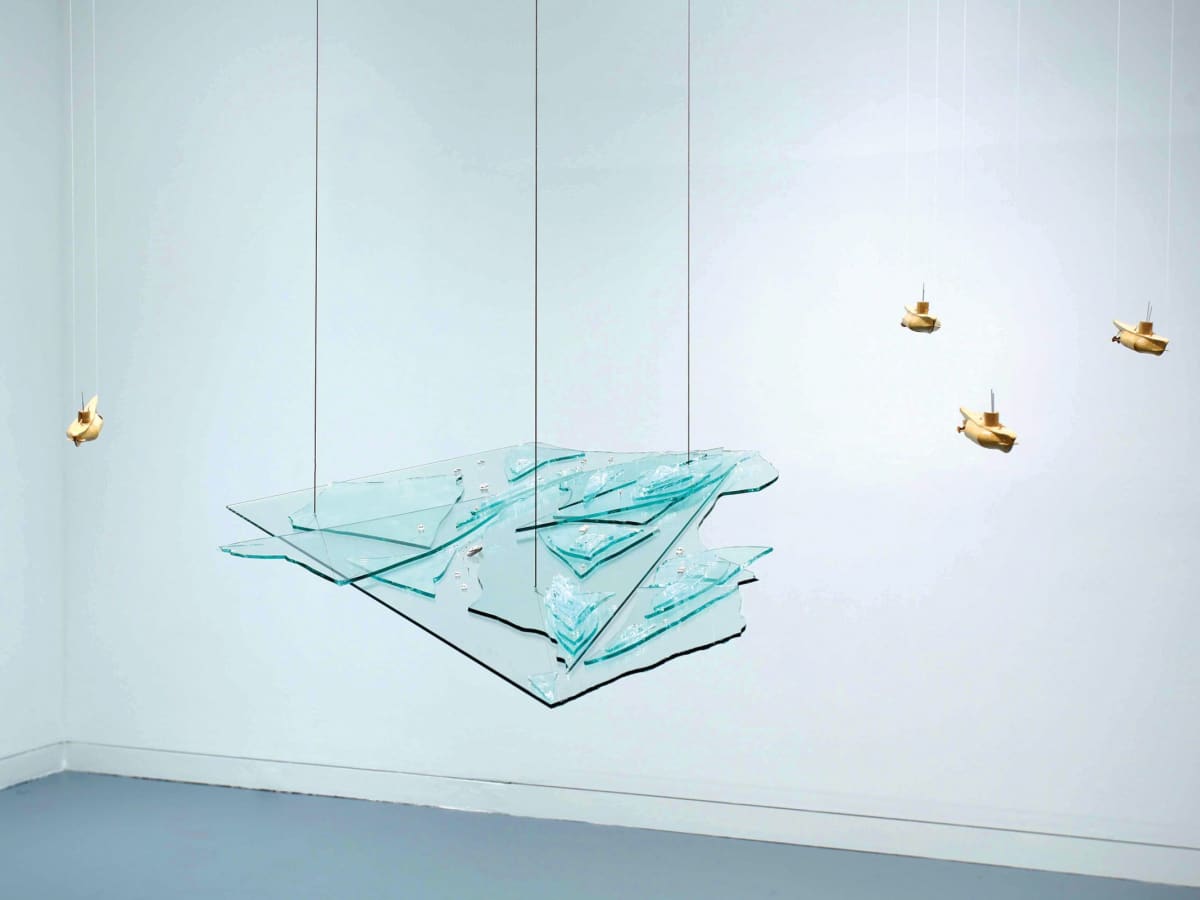This wide rectangular photograph captures an indoor scene of an art exhibit, likely within an art museum. The floor at the bottom of the image is a bluish-gray, tilting slightly upward from right to left. The background wall is a light gray with a subtle bluish tint. On the left side, a small yellow boat-like object hangs from the ceiling by two thin white strings. Dominating the center is a striking large glass sculpture, composed of two bent almost square-like pieces of glass adorned with turquoise-colored shards, all held together by three vertical black cords. The sculpture, reminiscent of a fragmented map due to its intricate twists and turns, creates a focal point in the exhibit. To the right of this central piece, near the top right corner, are three more yellow plastic boat-like objects, each suspended by two white strings, adding balance and additional interest to the visual composition.